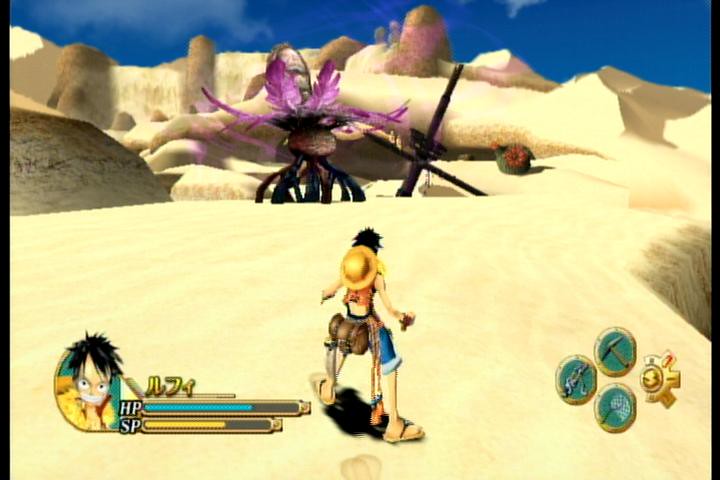This image captures a scene from a cartoon-styled video game set in a desert environment. The upper part of the image features a clear blue sky, with a touch of cloud coverage on the left side. Below, the landscape unfolds into a vast, sandy expanse with undulating waves of sand. A prominent rock sculpture, light brown with darker brown hues on top, dominates the left side. Transitioning to the right, there are two smaller rocks followed by another elongated rock structure.

Near the center, slightly to the left and slightly elevated, stands a distinctive plant resembling a turnip. This plant has large, purple leaves and exposed black roots extending into the sand. Below it lies a brown, round object. 

To the immediate right, the mast of a boat ascends diagonally, accompanied by a horizontal cross-beam. Behind the mast is another large rock formation tinged with brown and hints of pink. Adjacent to the mast, a small green pot with a flower adorns the sand.

Center-stage, a character stands with his back turned. He is wearing a yellow straw hat, a red vest, short blue jean shorts, and brown flip-flops. He carries a small bag hanging from his waist. This character, Monkey D. Luffy from the manga 'One Piece,' is depicted with black hair. 

The gaming interface is evident: the bottom left features the character's avatar and health bar, with HP displayed in teal and SP in yellow. The bottom right corner shows four circular icons, including a pickaxe, grappling gun, net, and a compass.